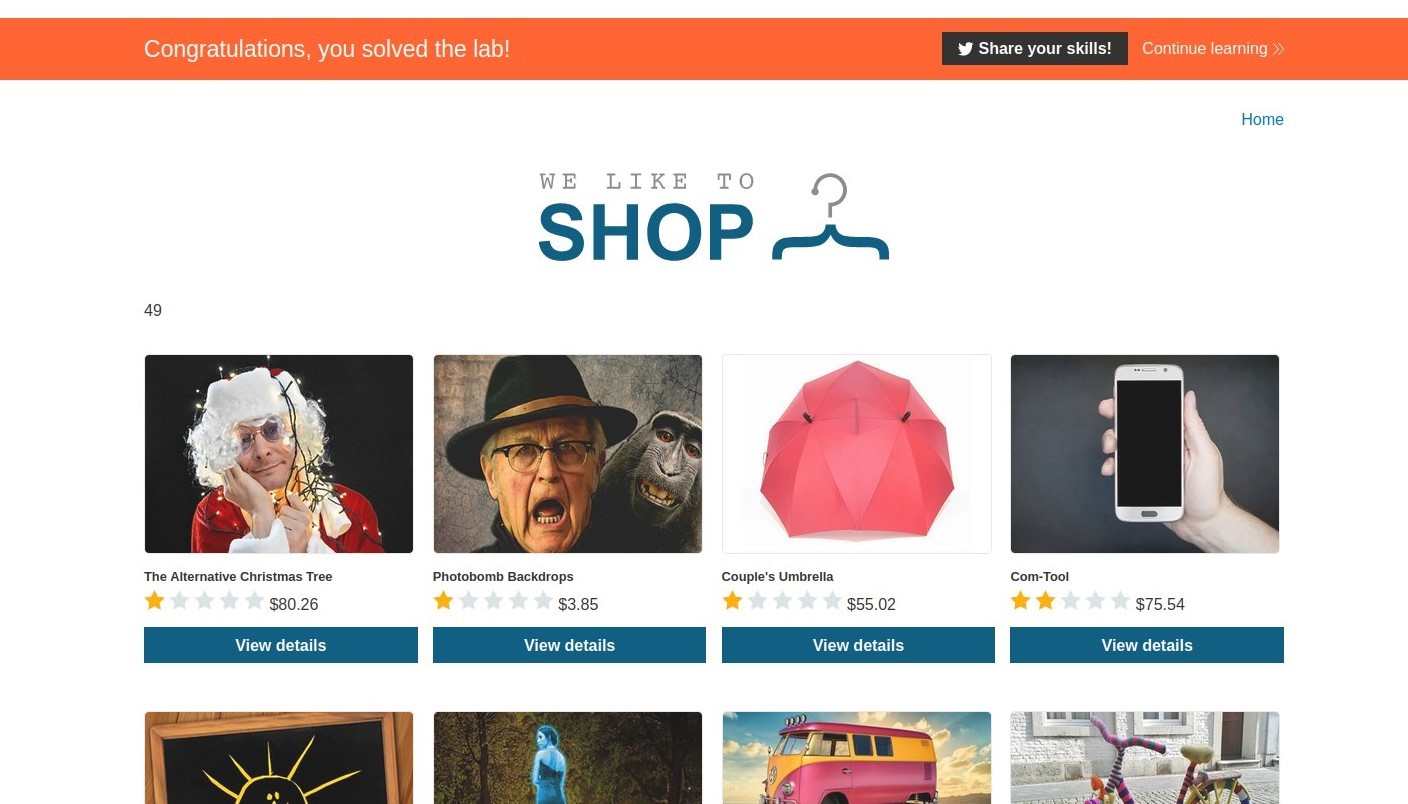The screenshot captures a congratulatory message from a website, set against an orange background with white text at the top reading, "Congratulations, you solved the lab." Below this message, there is a button featuring the Twitter logo and the text "Share your skills," followed by another button labeled "Continue Learning."

Further down, an image displays text that reads, "We like to shop." This image is creatively designed to show a hanger, cleverly composed of a combination of a question mark and a text bracket. Below this, there is a series of product images available for purchase. Each product is rated with stars: most have one star, except for one which has two.

The products listed are:
1. **The Alternative Christmas Tree** - $80.26
2. **Photobomb Backdrops** - $3.85
3. **Couple’s Umbrella** - $55.02
4. **Comm Tool** - $75.54 (this item has two stars)

There are an additional four images of items below these, but the text descriptions for these are not readable.